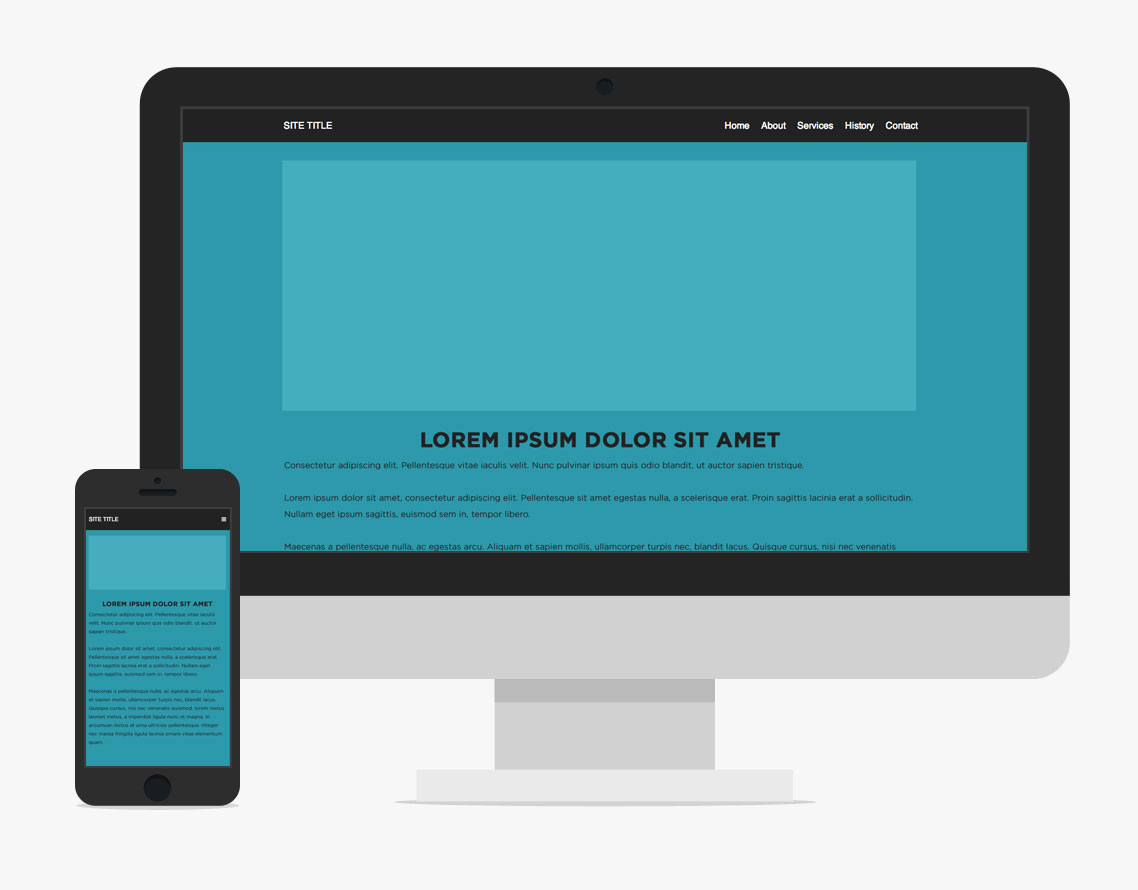In the generated image, a black smartphone and a computer monitor with a black frame and white bottom border and base are featured side-by-side. Both devices display the same blue-themed website page titled "lorem ipsum dolor sit amet" with white menu items, including site title, home, about, services, history, and contact. The phone, presenting the content in a mobile format, mirrors the website on the computer screen, down to the foreign language text at the bottom. The monitor's black upper border frames the site content, matching the aesthetic of the smartphone's display.